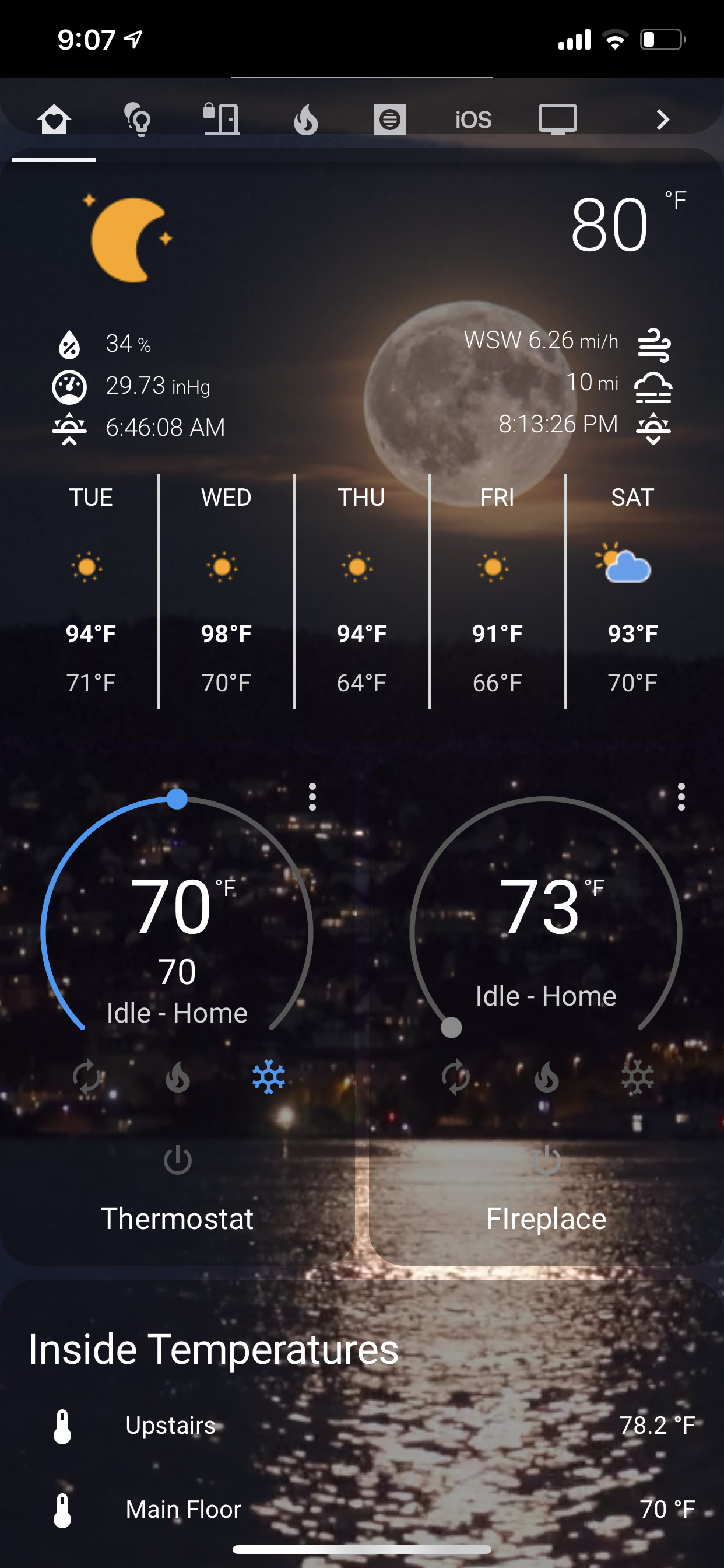Screenshot of a mobile device captured at 9:07 PM with a predominantly black background. The device shows four bars of cellular service and two bars of Wi-Fi with the battery level at approximately 30%. This iOS device is displaying a weather app. On the left side of the screen, an icon of a moon indicates nighttime, with the temperature reading 80°F on the right side. Additional details include current pressure, sunrise, and sunset times. The app also displays a five-day forecast, indicating that from Tuesday to Saturday, temperatures will reach the 90s during the day and drop to the 60s or 70s at night. Also visible in the screenshot are the home automation settings: the thermostat set to 70°F while the home is marked as idle, and an adjustable fireplace setting.